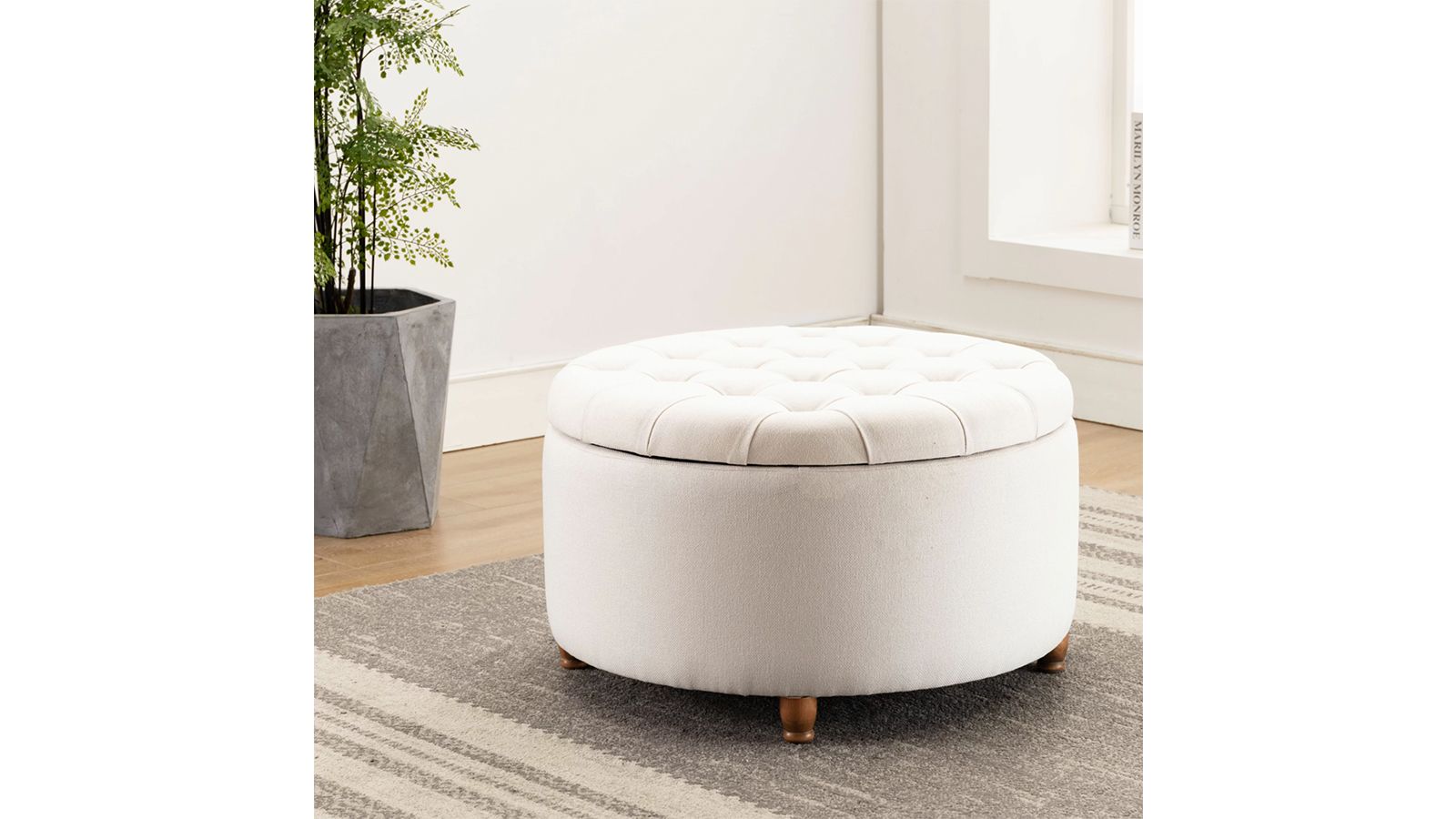This full-color photograph captures a meticulously arranged indoor scene, likely taken on a sunny day. Dominating the center of the square image is a white, round ottoman with small wooden legs, the top of which appears to be removable for storage purposes. This ottoman rests on a gray rug adorned with white stripes, which, in turn, is placed atop a light brown wooden or laminate floor. To the left, a gray vase with a triangular pattern houses a lush green plant, adding a touch of nature to the setting. The backdrop features white walls and, in the upper right corner, light streams through a window with a wide sill. Additionally, there's an unidentifiable, small word running along the right side, enhancing the meticulous details captured in this photo.